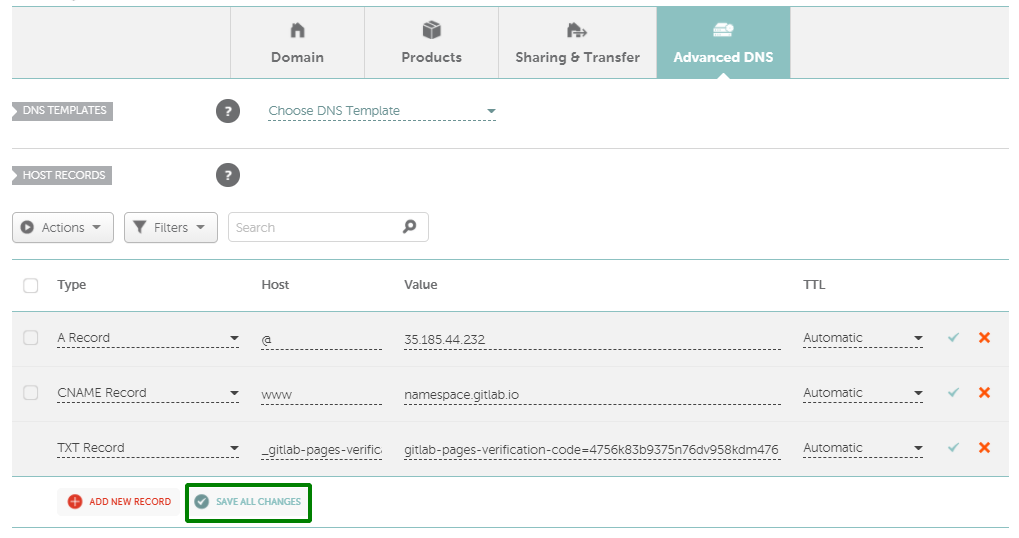The image displays a website or application interface primarily featuring a white background with gray sections and black text. At the top of the interface, there is a gray navigation bar with multiple sections labeled "Domain," "Products," "Sharing and Transfer," and "Advanced DNS," with the "Advanced DNS" section highlighted in green. 

Beneath this navigation bar, there is a section titled "DNS Templates," accompanied by a question mark icon, providing the option to choose a DNS template via a clickable button. Below the "DNS Templates" section, another section is labeled "Host Records," also accompanied by a question mark icon. This section features two buttons labeled "Actions" and "Filters," alongside a search box for easy navigation.

Further down, there is a detailed display of DNS records grouped in a table. The table columns are labeled "Type," "Host," "Value," and "TTL." The three DNS records listed include:
1. **A Record**: Host is "@", Value is "3.5.3.8185.44232", and TTL is set to "Automatic".
2. **CNAME Record**: Host, Value, and TTL details similar to the first record.
3. **TXT Record**: Host, Value, and TTL details similar to the first record.

Each record in the table ends with two icons: a check mark and an X, presumably for approval and deletion, respectively, indicating actions that can be taken on each DNS record.